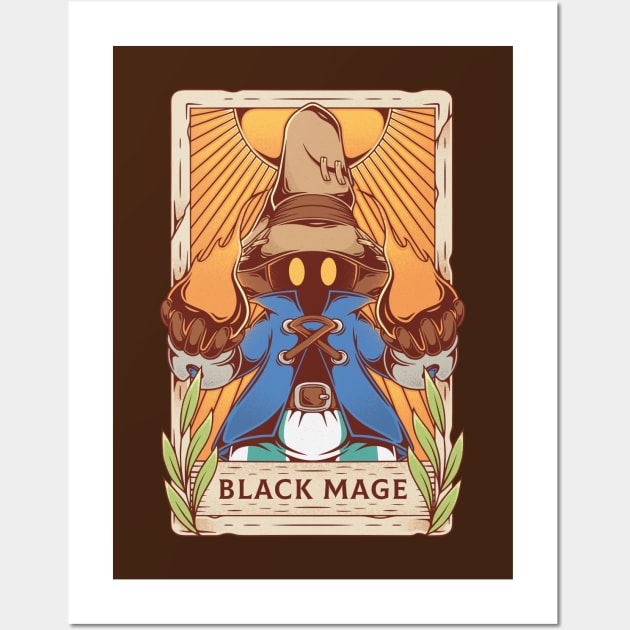This image is a detailed poster-style graphic design resembling a trading card. Set against a black background, the centerpiece features a character labeled "Black Mage" in text bordered at the bottom, flanked by green leaves resembling high grass. The central figure, described as a shaman or fantastical mage, has a black face with striking yellow eyes, wearing a large brown hat with a belt and clip. Dressed in a blue cloak with crisscross strings, a brown belt, and striped blue and white pants, the character holds flames in both gloved hands. A bright orange sun blazes behind him, adding a dramatic flair to his imposing, magical presence.